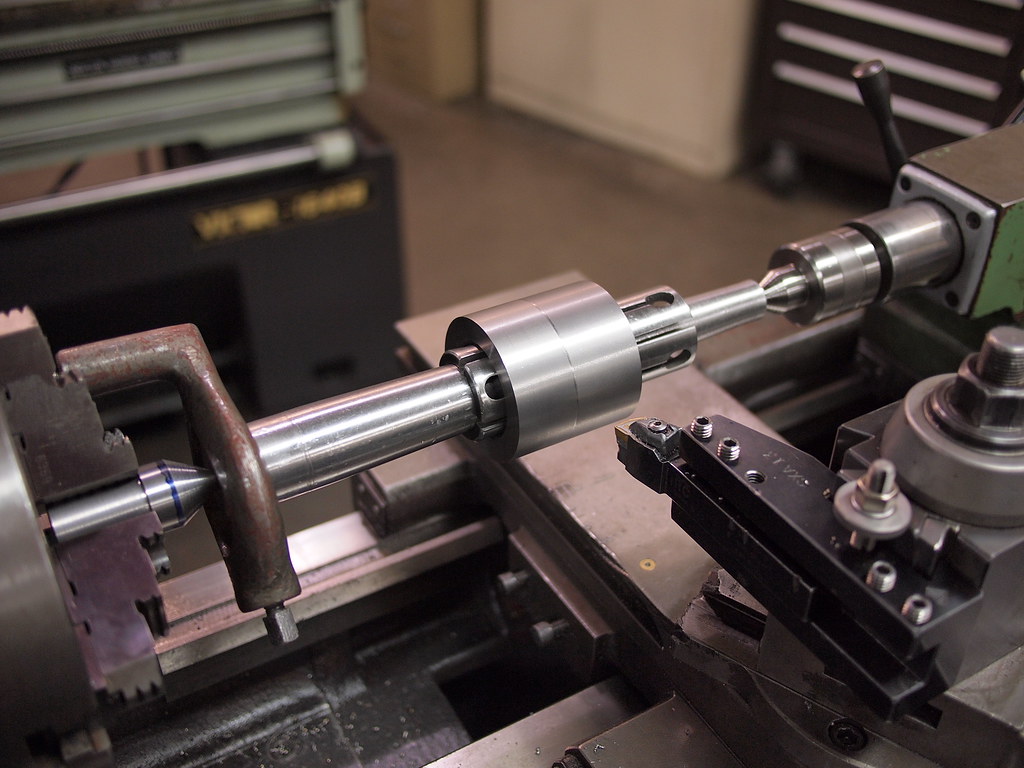A close-up, highly detailed photograph captures a vintage piece of industrial machinery, resembling a horizontal drill press. The machine, bathed in the iconic green paint commonly found on mid-20th-century manufacturing equipment, features a prominent lever at the rear. Dominating the frame is a shiny stainless steel component, perhaps an injector arm or another precision part, contrasting with the green casing. This particular piece, either a part of the machine or its manufactured output, hints at varied possible uses—ranging from automotive pistons to components of complex systems. In the blurred background, a utilitarian gray concrete floor and cabinetry can be observed, including a machinist's tool cart with broad, metal pull-out drawers, suggesting the setting of a well-equipped workshop.